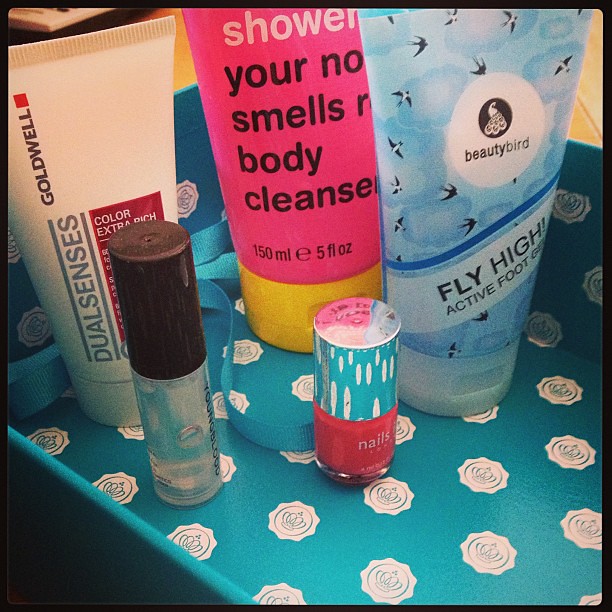The image depicts a close-up of a blue tray adorned with white flower-shaped patterns, each featuring a crown inside. Arrayed neatly on the tray are five distinct beauty and hygiene products. In the back row, there are three tubes: a white tube on the left labeled "Goldwell Dual Senses Color Extra Rich," a central pink tube with a yellow cap labeled "Shower Your Smells Body Cleanser," and a white tube with blue patterns on the right labeled "Beauty Bird Fly High Active Foot." The front row features two smaller cylindrical bottles: a transparent serum with a white cap on the left, and a red nail polish with a yellow and silver cap on the right. The blue tray and its assorted products create an organized display, emphasizing both skincare and beauty items.